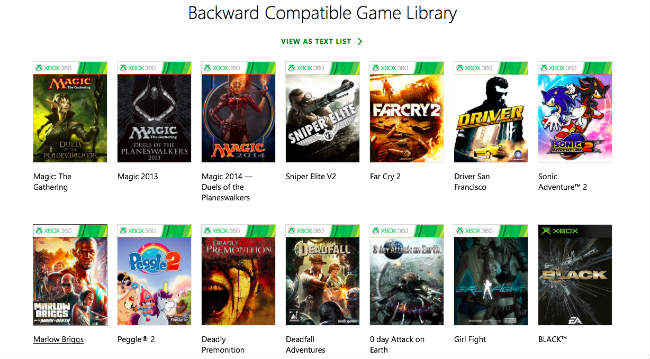This image showcases a web page interface on an Xbox console, specifically displaying the user's game library of previously purchased titles. The header of the page has "Backward Compatible Game Library" written in black text. Below the header, there's an option highlighted in green labeled "View as Text List." The games are organized into two rows, each arranged from left to right. 

In the top row, the first game listed is "Magic: The Gathering," followed by "Magic 2013," "Magic 2014: Duels of the Planeswalkers," "Sniper Elite V2," "Far Cry 2," "Driver: San Francisco," and "Sonic Adventure 2." 

The bottom row begins with "Marlo Briggs," followed by "Peggle 2," "Deadly Premonition," "Deadfall Adventures," "Zero Day: Attack on Earth," "Girl Fight," and lastly, "Black." Note that the text is somewhat unclear, making some titles appear fuzzy.